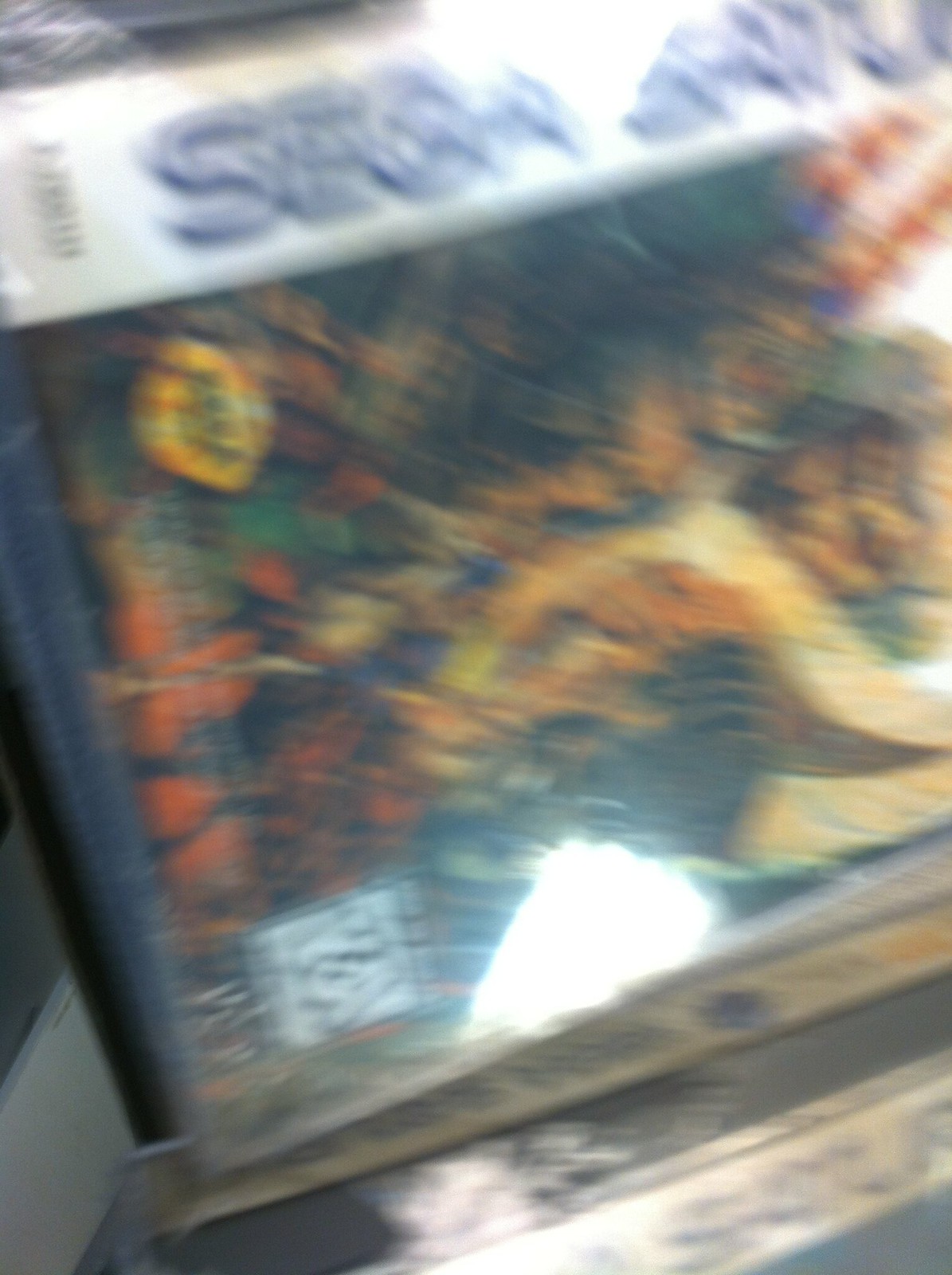This is an extremely blurry, low-resolution photograph of a SEGA video game case, captured at a poor angle. At the top of the image, "SEGA" is prominently displayed in blue letters against a long white stripe. The plastic case reflects light from either an overhead source or the camera flash. The front cover is obscured, hiding the specific game it contains, though the intricate illustration features colors like orange, green, yellow, red, white, and tan that suggest a possible creature or complex design. The case stands upright, and although the background is difficult to discern, there appears to be another identical game case underneath it. The overall image is difficult to interpret due to the combination of blur and poor angle.